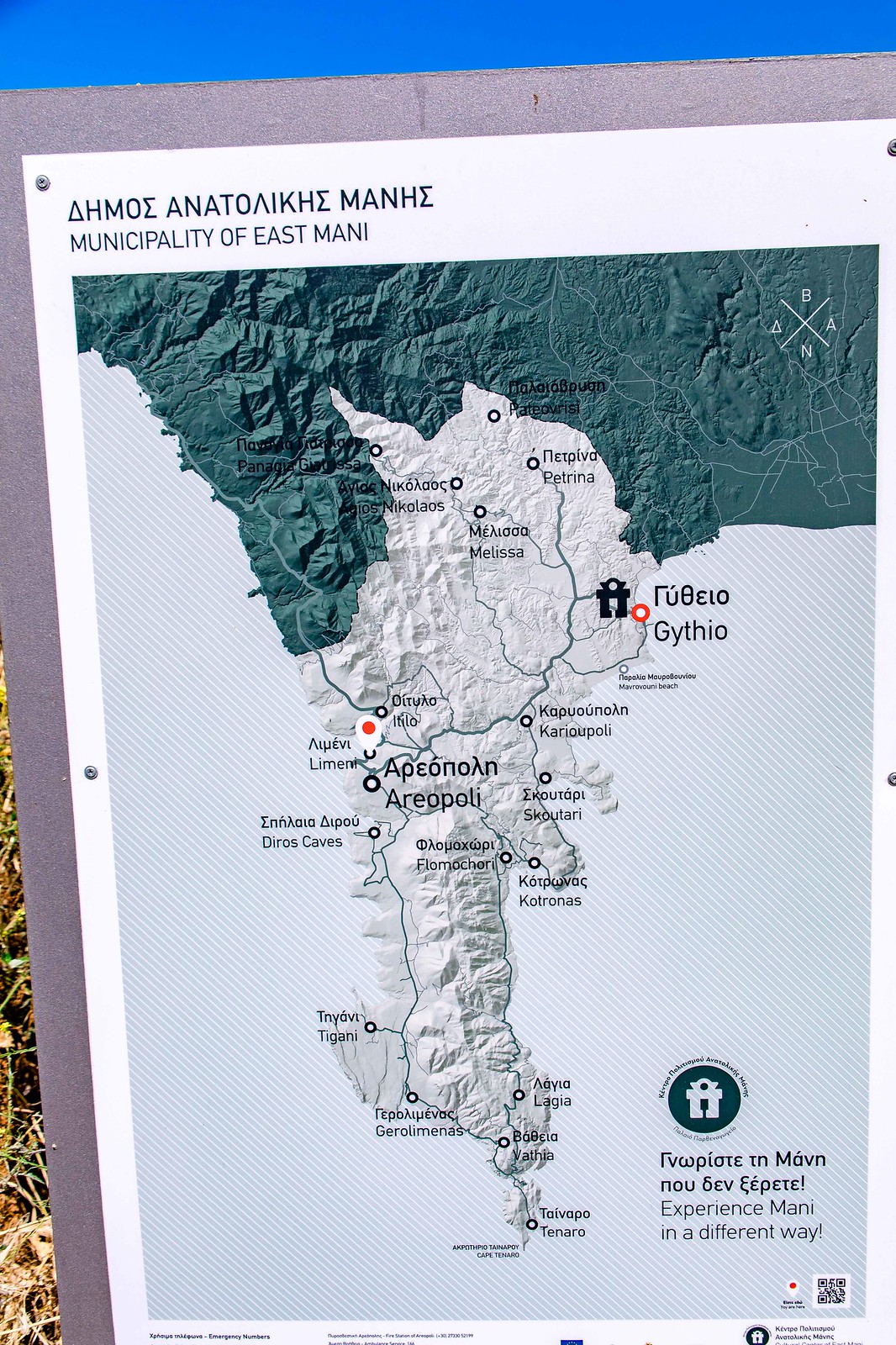The image depicts a map set up on a sign located in a grassy, wooded area. The map, which appears to be of a region labeled 'municipality of East Manny', is presented on a white piece of paper tacked to a gray board. The map features two prominent red dots, likely representing the capitals Githio and Arepilli. While the main text is in a foreign language, possibly Greek, there are some English phrases visible, such as 'Experience Manny in a different way.' Notably, the map itself has silver and gray landmasses and a light blue background. At the bottom right-hand corner, there is a logo resembling a gift box followed by Greek text. Overall, the sign seems to function as an informational guide, probably situated within a national park or a similar venue, aimed at helping visitors navigate the area.